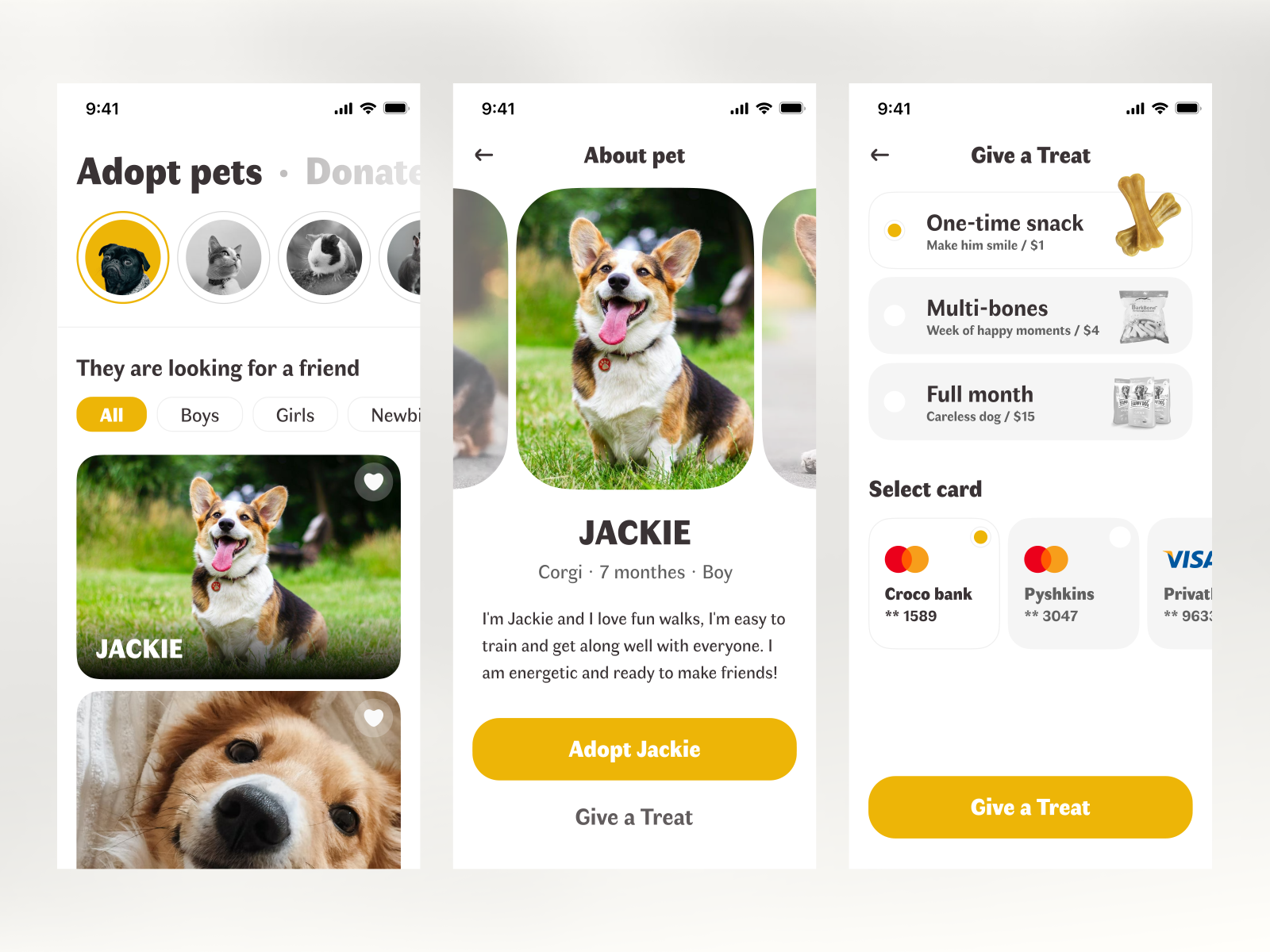Here is the descriptive caption for the series of screenshots:

---

This image consists of three overlaid screenshots on a white-gray background. Each screenshot features the same status bar icons at the top, indicating the time as 9:41, along with the Wi-Fi signal, cellular signal strength, and a fully charged battery symbol.

The first screenshot displays an interface titled "Adopt Pets" with a grayed-out "Donated" option. Below the title, there is a series of circular images of various animals. The first image is of a black pug within a gold circle. Following it are three images in gray: a cat gazing sideways, a hamster or rodent, and a partially visible image of potentially a bird. Under these images, the text reads "They are looking for a friend." The interface allows sorting options with tabs labeled "All," "Boys," "Girls," and "Newbies" in gold and white. The page lists pets, starting with an entry for "Jackie," accompanied by a picture of a tan, black, and white dog with its tongue sticking out, sitting on grass. A white heart icon is present in the corner of Jackie’s photo. Another dog photo below shows a light blonde fluffy dog with black eyes and a black nose, seemingly asleep on a white soft surface, also marked with a white heart icon.

The center screenshot features the interface for "About Pet." It showcases a back arrow and repeats the status bar icons. The highlighted pet’s name, "Jackie," is detailed as a "Corgi, seven months, boy." The description reads: "I'm Jackie, and I love fun walks. I'm easy to train and get along well with everyone. I am energetic and ready to make friends." Below the description is a button in white and gold labeled "Adopt Jackie," with a grayed-out "Give a treat" button beneath it.

The last screenshot is from the "Give a Treat" section. Mirroring the prior status bar icons and back arrow, this screen displays treat options. The first option, labeled "One-Time Snack, Make him smile," features rawhide bones and is priced at $1. The next two options are grayed out: "Multi-Bones, Week of happy moments" for $4 with a picture of a dog treat bag, and "Full Month, Careless dog" for $15 with several treat bags. At the bottom, there is a section to "Select Card," displaying payment methods including two MasterCard logos ("Crocco Bank" ending in 1589, and "Sykins" ending in 3047), and a partially visible Visa card ("Private" ending in 963). A gold and white button at the bottom right says "Give a treat."

---

This caption provides a comprehensive description of the screenshots, detailing the content and visual elements thoroughly.